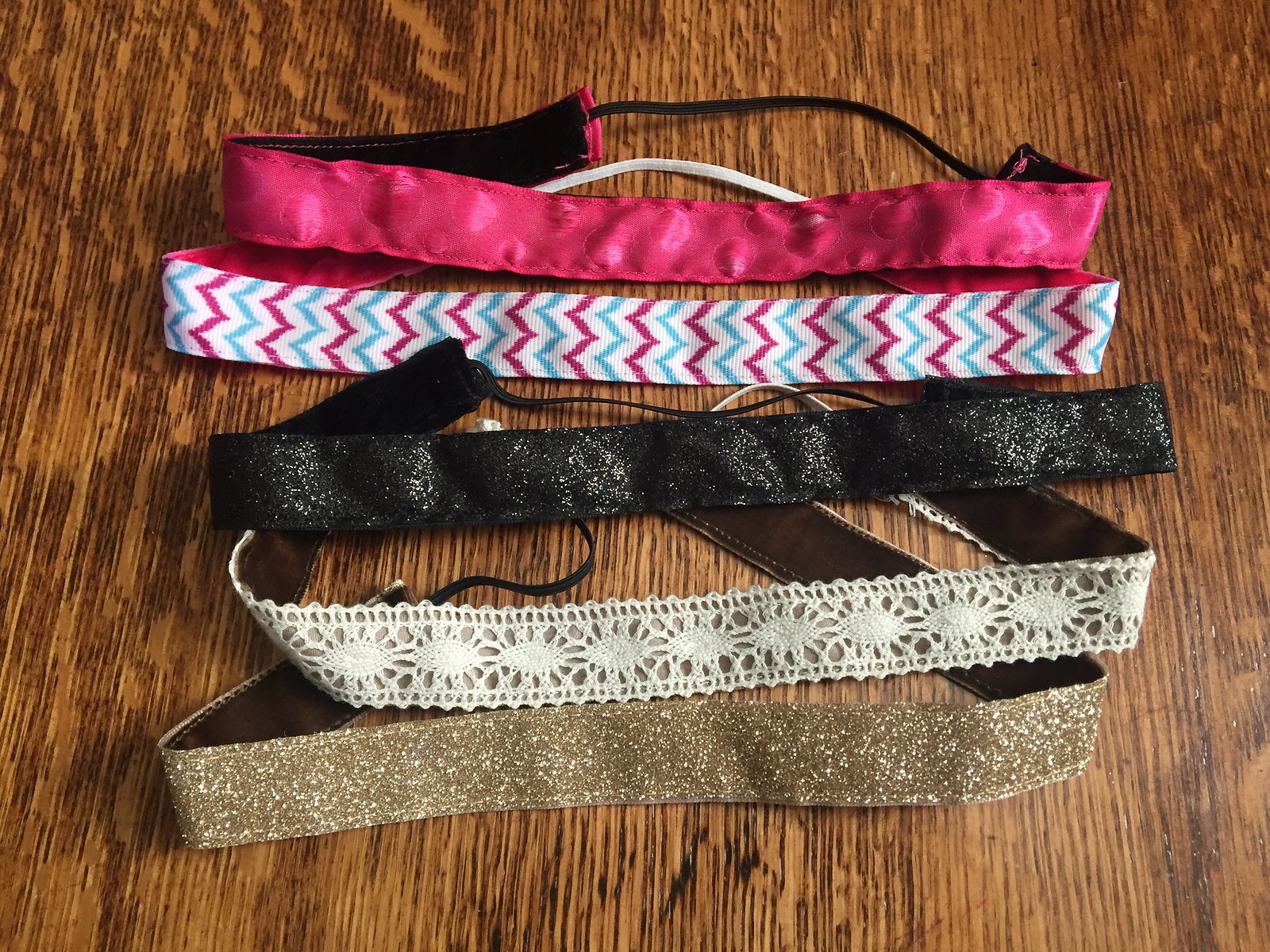Displayed on a dark brown wood grain table, running vertically are four headbands designed to hold hair back. The table's rich brown surface features distinct vertical grains. Arranged diagonally from top left to bottom right, the headbands are spaced evenly with about an inch distinguishing them on either side. 

The first headband at the top showcases a bright pink exterior with a visible black interior, connected by a black string. Below it, the second headband prominently features a white background adorned with zigzag stripes in purple and blue. The underside of this headband is dark pink, and it also features a connecting string. 

Further down, the third headband is entirely black, including its connecting string, giving it a uniform, sparkling appearance. The fourth headband stands out with a white, doily-like pattern suggesting a knitted or crocheted texture; its underside is brown, and it is held together by a white string. 

Finally, the fifth headband at the bottom has a brown and gold sparkling exterior, with the underside and string both black, completing this diverse and colorful arrangement.